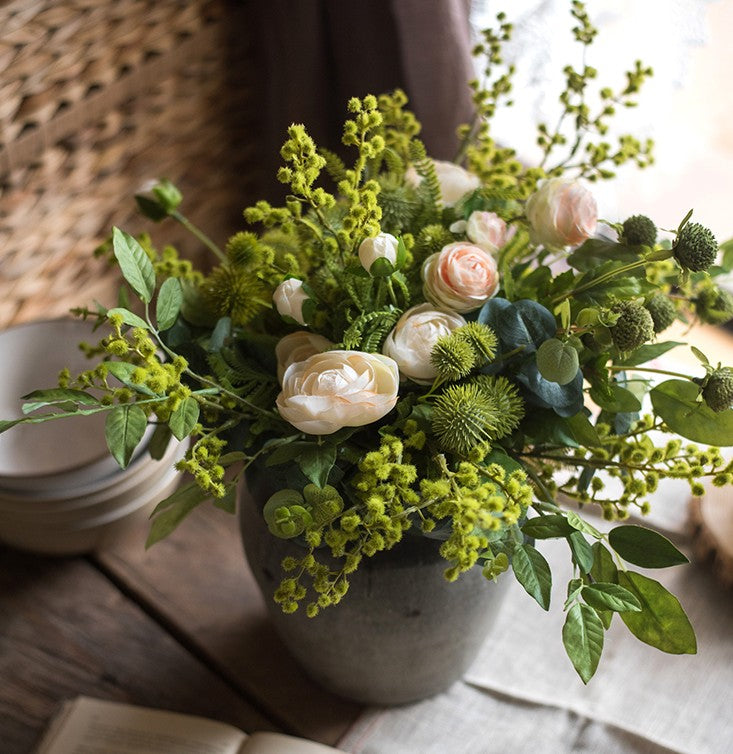The image showcases a gray-and-black clay pot filled with an assortment of vibrant plant life, prominently featuring light pink and white roses alongside various green foliage. Among the greenery are leaves, soft green ball-like flowers in different sizes, and touches of fern. This pot rests on a dark wooden table, partially covered by a light brown napkin. Beside the arrangement, there are stacked light brown bowls and an open book. The background reveals what appears to be wicker furniture or a wicker-textured wall, highlighted by sunlight streaming through a nearby window, illuminating the scene.